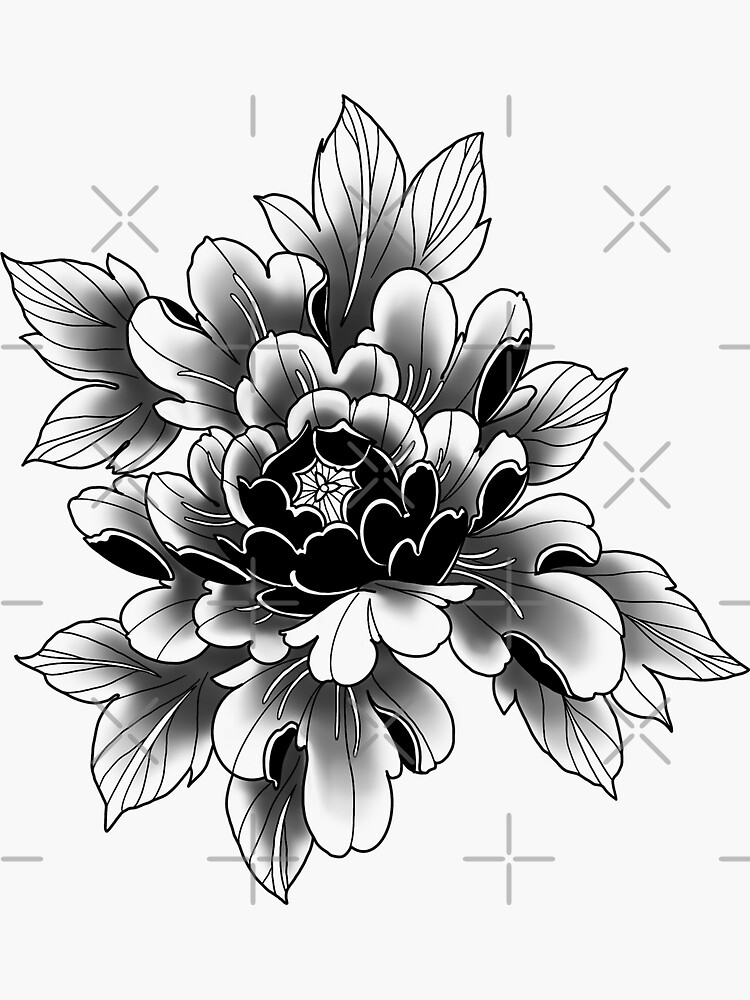The image depicts a detailed black and white graphic artwork of a flower, which closely resembles a chrysanthemum. The composition is presented in portrait orientation, featuring a blooming flower with an intricate design against a clean, pure white background. Central to the flower is a three-sided triangular shape surrounded by tightly packed lines that gradually loosen as they extend outwards. The flower is adorned with numerous petals, too many to count, and encompasses leaves with white interiors and black exteriors. Additionally, there are multiple crosshairs crisscrossing the image, forming a pattern of alternating plus signs and X’s, likely serving as watermarks. The overall aesthetic captures a blend of artistic detail and symmetry, making it reminiscent of a tattoo template or stock art.